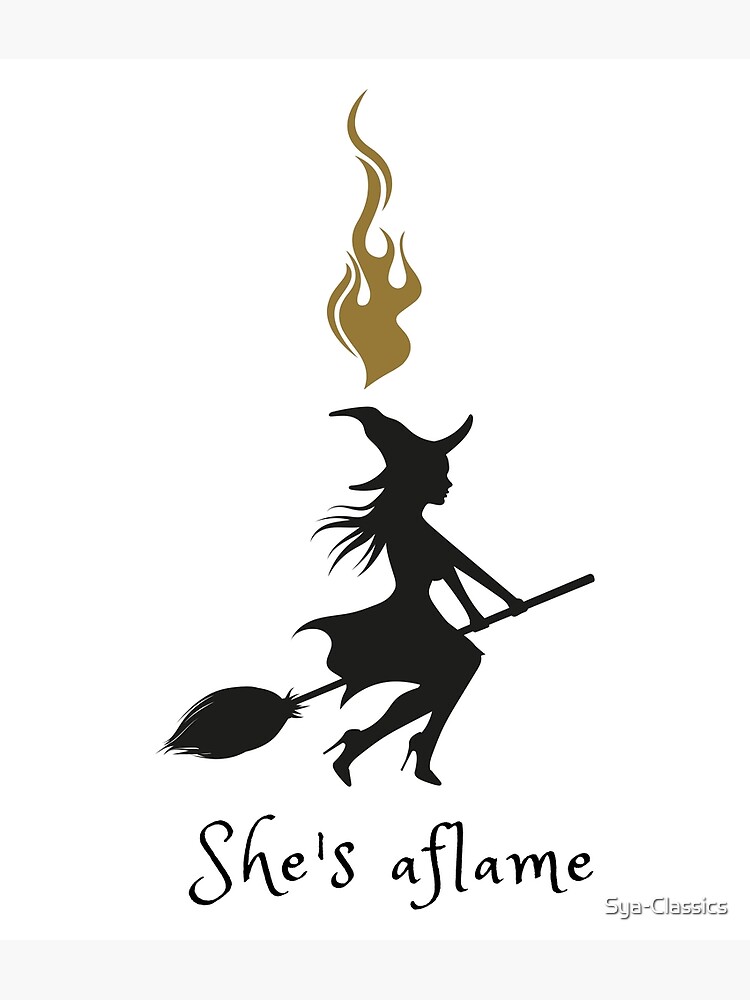This image features a traditional, silhouette-style depiction of a witch riding a broomstick. The witch is dressed entirely in black, with a pointed hat and high heels, creating a striking contrast against the white background. Her hair is flowing behind her as if caught in the wind, and she grips the broom with both hands. Above her head, a golden flame rises, adding a touch of vibrant color to the monochrome scene. Beneath the witch, the text "She's a Flame" is written in an ornate, curly font. In the lower right corner, there is a watermark reading "S-Y-A Classico" in light gray lettering. This detailed logo blends classic witch iconography with modern, minimalist design elements.